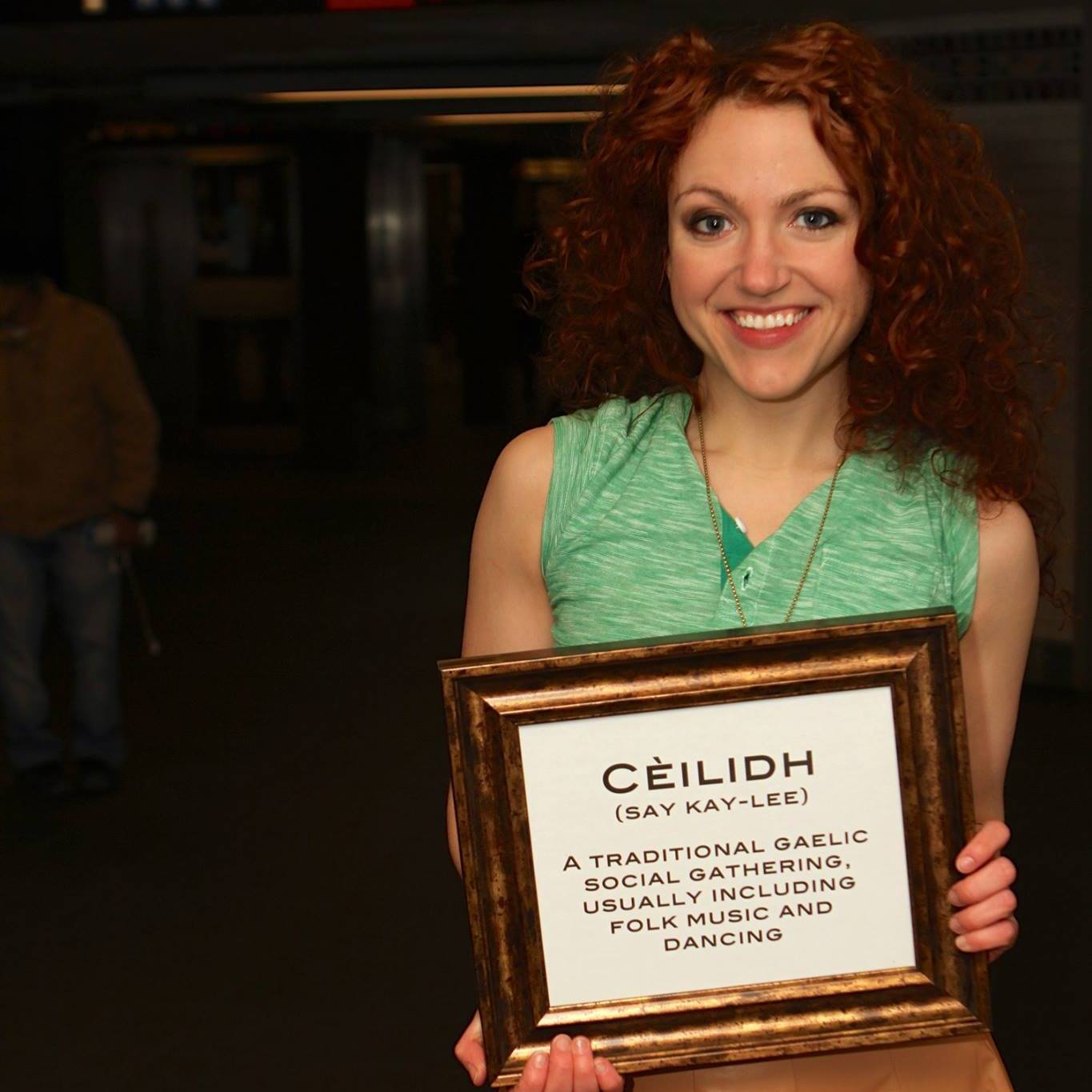In this detailed zoomed-in image, we see a front-view portrait of a woman proudly holding a framed certificate. She is wearing a green shirt and has long brown hair cascading over her shoulders. The woman is smiling warmly, exuding a sense of accomplishment. Her left hand, positioned towards the lower part of the frame, reveals four fingers while her thumb rests in the background. Similarly, her right hand grips the right edge of the frame, displaying four fingers.

The frame she is holding is square-shaped, a dark brown hue adorned with light brown accents. Encased within the frame is a white square featuring black text. The inscription reads: "Céilidh (Kaylee): A traditional Gaelic social gathering, usually including folk music and dancing."

The background is entirely black, which enhances the focus on the woman and her certificate, isolating them as the central elements of the image.